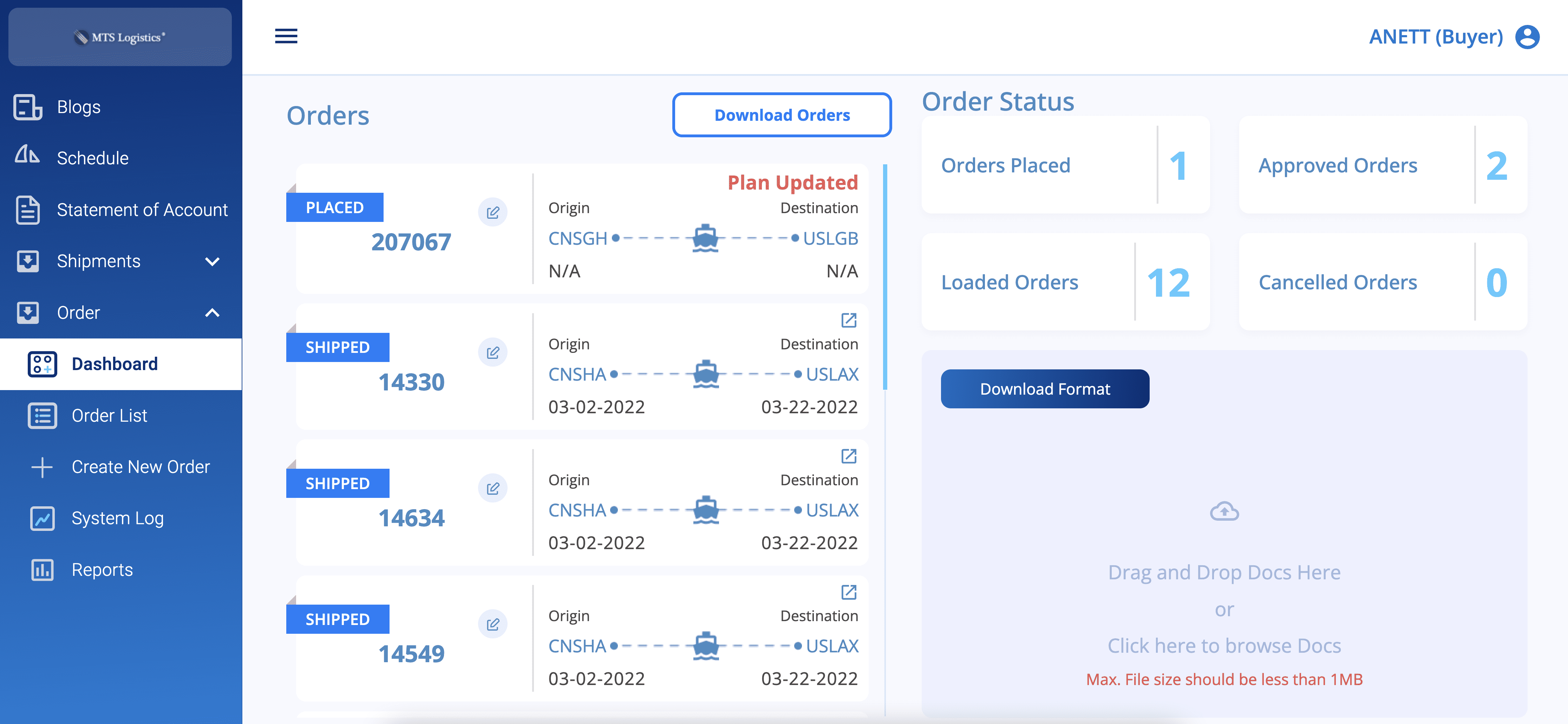Detailed Caption: 

The image is a screenshot of an order dashboard from MTS Logistics, showcasing a buyer profile, presumably belonging to an individual named Annette. The interface features a navigation menu on the left-hand side, listing options such as Blog, Schedule, Statement of Account, Shipments, Order Dashboard, Order List, Create New Order, System Log, and Reports.

The main dashboard area is primarily focused on order management. It displays detailed information on various orders, including their current status. Each entry provides an order number, the origin code, and the destination code, with the respective dates listed beneath. 

To the right, the dashboard categorizes orders by their status – placed, shipped, approved, loaded, and canceled. Users are also given options to download data in a drag-and-drop format, further streamline the process.

The entire dashboard is designed in a clean, blue and white color scheme, enhancing readability and user experience.